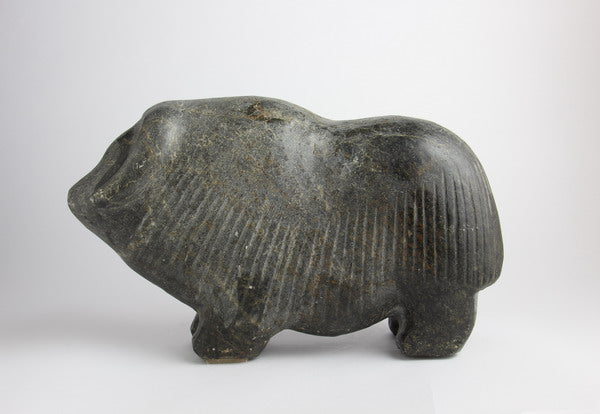This image depicts an ancient, weathered stone figurine set against a white background. The figurine, seemingly carved from a grayish-black marble or rock, resembles a bulky animal like an elephant or rhinoceros, though its exact identity is ambiguous and uncertain. Notably, the figurine lacks a discernible head, presenting instead a rounded, swirly area at the front, possibly the rim of a cavity or mouth. The body of the creature features a series of thin horizontal indentations, in contrast to the smoother top that reflects a white light source. The sculpture stands on four short, stumpy legs, without visible claws or paws. Despite signs of erosion and wear, hints of lighter beige in the indentations and shadows suggest the details of age and craftsmanship.